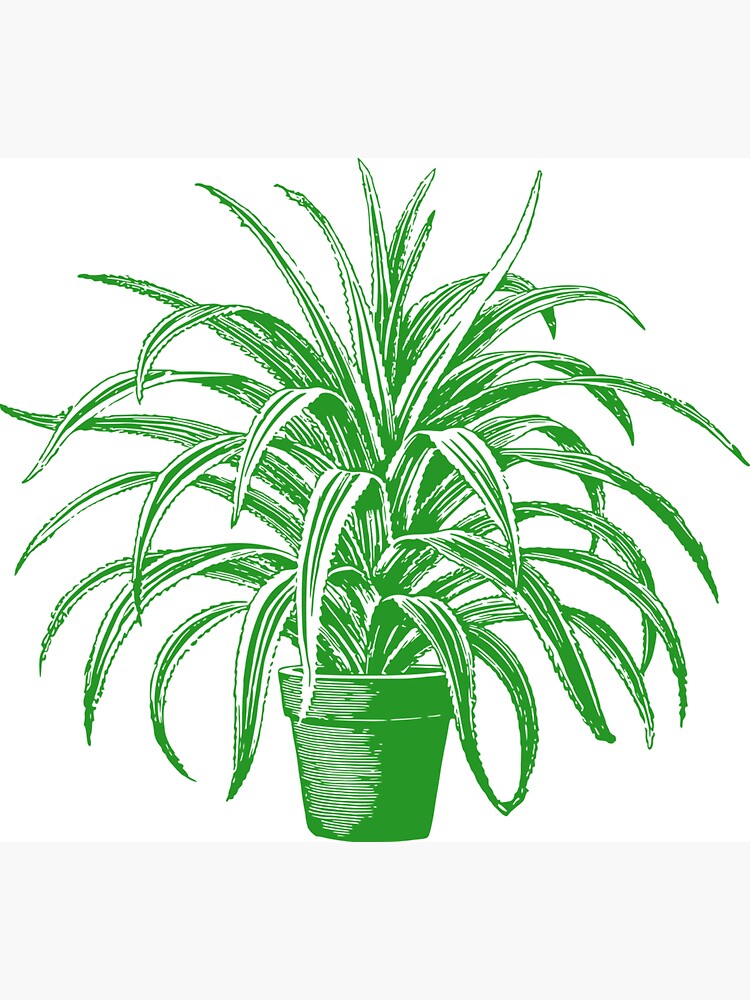This is a detailed representational illustration of a plant that closely resembles a spider plant or an elephant ear plant. The plant, which is depicted with long, green fronds accented by white stripes, somewhat resembles the top of a pineapple on steroids. The leaves are numerous and layered, with some standing upright while others cascade downwards, almost touching the ground. The pot, a standard red clay design, contains this voluminous mass of foliage, adding to the lively and textured look of the plant. The pot itself features a two-tone shade of green with solid areas interspersed with white lines, suggesting motion or texture. The illustration has a professional finish, possibly using watercolor or another design format, and is set against a simple white background, highlighting its botanical garden-like quality.